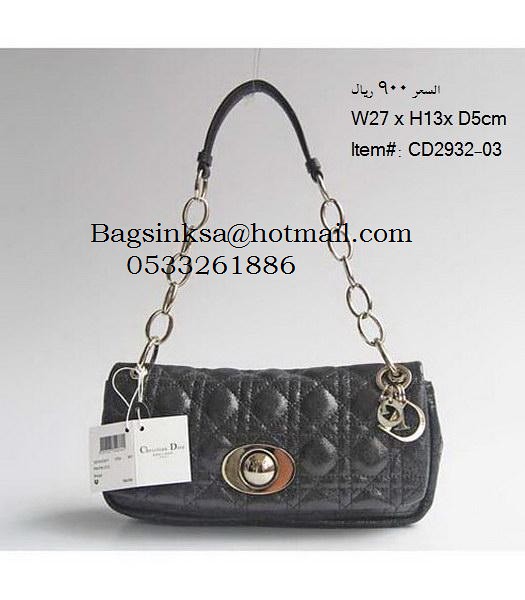This is an image of what appears to be a knockoff Christian Dior black quilted leather pocketbook. It is rectangular and relatively small in size, with noticeable circular and triangular textures. The bag features a gold clasp in the middle and a metal chain handle with a leather section at the top for comfort. Hanging from the bag are charms that spell out "CD."

On the left side of the strap, there is a tag that says "Christian Dior," and on the right side, it has the "CD" charms. The image has a white border and a gray background. An email address "bagcincsa@hotmail.com" and a phone number "05-332-61886" are overlaid on the bag, indicating it's likely being sold online. Additionally, the phrase "Bags Inc. Sa" is present. 

The item dimensions are specified at the upper right-hand corner in both English and Arabic: W27 x H13 x D5 centimeters, and the item number is CD2932-03. Despite the detailed specifications provided, the overall presentation and the email address used suggest it might be a counterfeit product.